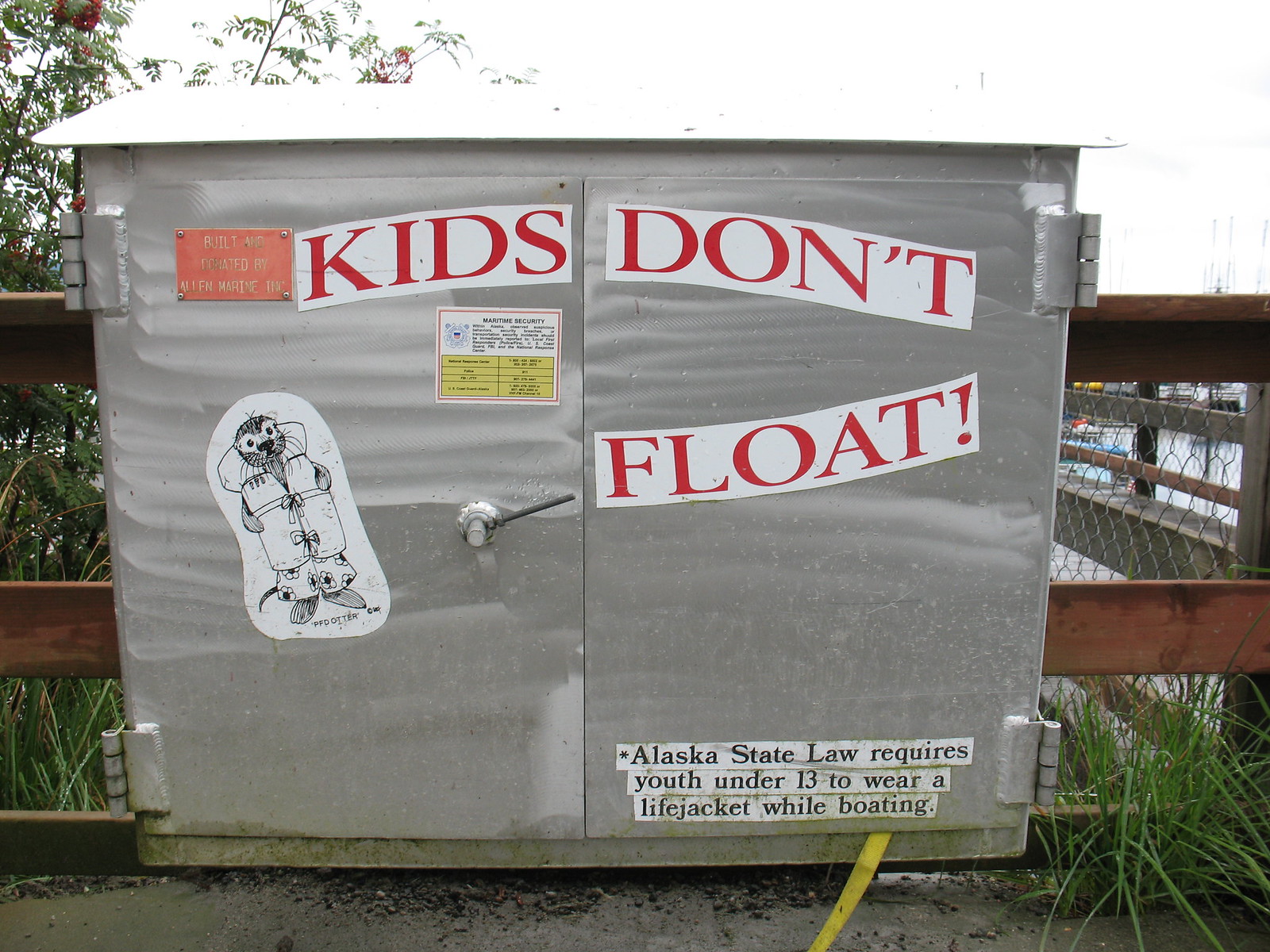The image features a stainless steel storage box mounted on a wooden railing along a dock, likely near a waterfront or harbor entrance. The box has two metal doors, each attached with welded metal hinges on either side, and a single latch on the left door. Prominently displayed across the front of the box are three large white stickers with red text, each containing one word: "Kids Don't Float." On the left door, there is a cartoon graphic of an otter standing on its hind limbs, wearing swim trunks and a life vest. Below this graphic, another sticker provides safety information in black text that reads: "Alaska State Law requires youth under 13 to wear a life jacket while boating." A strap hangs out from the bottom of the box, suggesting that it likely contains safety or rescue equipment, possibly flotation devices. The box serves as a reminder and enforcement of safety regulations designed to protect young individuals while boating.